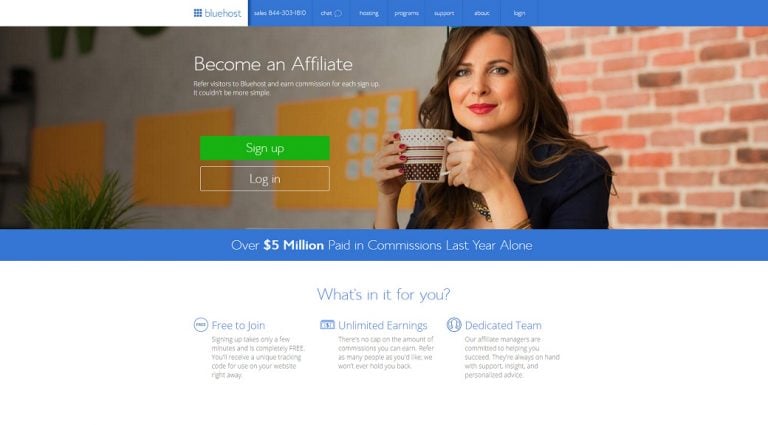This is a cropped screenshot of the Bluehost home page, specifically the affiliate section. Positioned towards the top left of the image is the Bluehost logo. To the right of the logo are seven categories: Chat, Pricing, Program, Support, Login, and others. 

Directly beneath this navigation bar is a large rectangular photo featuring a woman holding a cup of coffee. To the left of the woman, in large white font, the text reads "Become an Affiliate." Below this heading, additional information is presented in smaller white font.

At the very bottom of the image, there is a large green button labeled "Sign Up" and, directly underneath, a transparent button that says "Log In." 

Towards the bottom of the picture, a blue banner spans the width of the screen, with the text "Over $5 Million Paid in Commissions Last Year Alone." Centered beneath this banner, on a white background, is the text "What's in it for you." Following this, three examples are vertically aligned, detailing the benefits for affiliates.